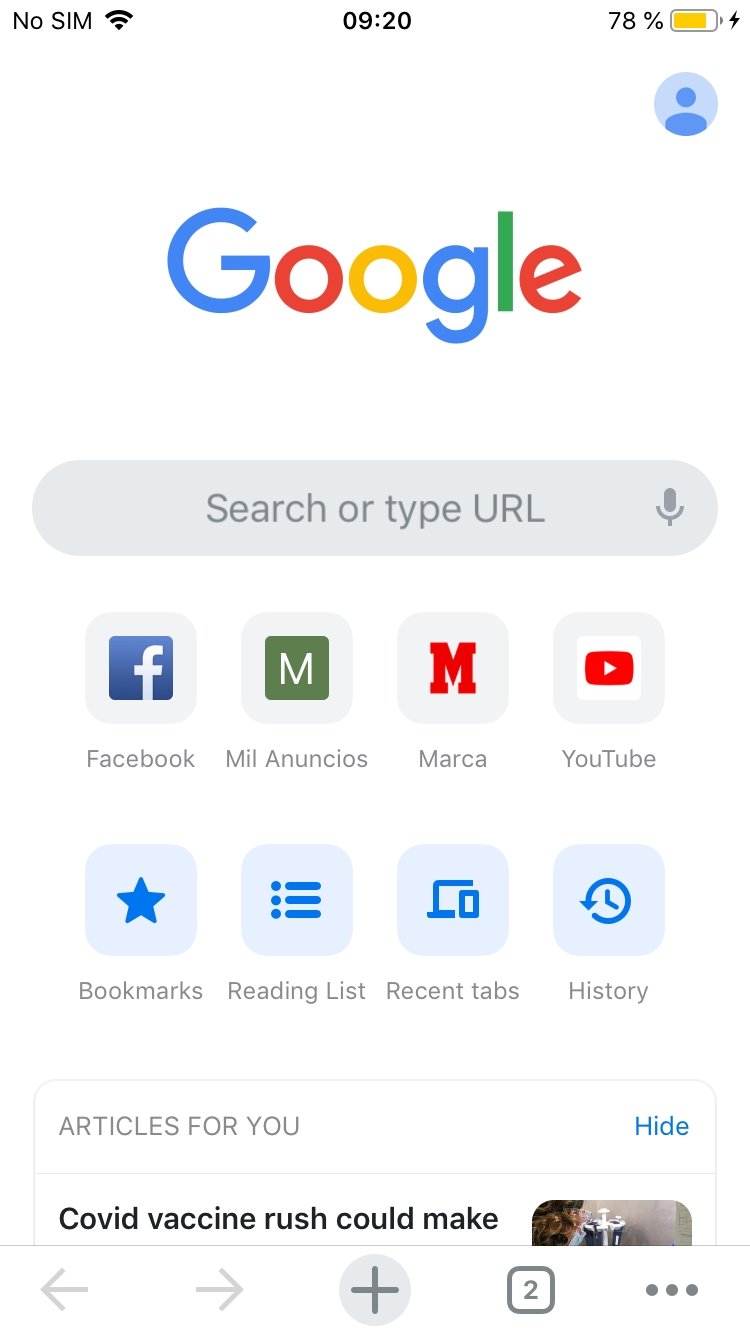In this image, we have a white background featuring various elements from a mobile interface. At the top, the status indicators display "No SIM," the time "9:20," and a battery level of "78%." Below this, there is a prominent blue circle icon with a small person inside it. Centrally positioned is the multicolored Google logo in blue, red, yellow, and green.

Underneath the logo is a blue search box. Below this search box, several light blue rectangular buttons are visible, each containing different items such as "Facebook," "Mil Anuncios," "Marca," "YouTube," as well as categories like "Bookmarks," "Reading List," "Recent Tabs," and "History."

Further down, there is another blue search box titled "Articles for You," with a "Hide" option on the right side. Partially visible beneath this box is the headline "COVID vaccine rush could make," accompanied by an incomplete image. A navigation bar at the bottom features a horizontal line, left and right arrows, a blue circle with a cross (possibly a close button), a square with a numeral "2," and an icon with three vertical dots, likely representing additional options or settings.